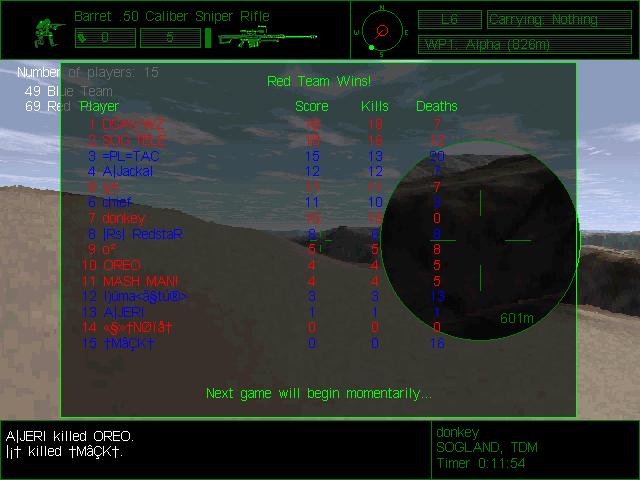The image is a screenshot captured during a video game session, primarily dominated by overlaid game information. In the upper left-hand corner, there is a detailed readout indicating the use of a Barrett .50 caliber sniper rifle, with a visible icon of the rifle accompanied by ammo status, showing 0 out of 5 rounds. At the top of the screen, the number of players is displayed as 15, along with the scores for the blue team at 49 and the red team at 69, indicating an ongoing competitive match. Central to the image is a bold banner announcing "Red Team Wins," accompanied by a list of game statistics such as kills, deaths, and other various scores, highlighted in red and blue fonts. Below these scores, a message informs the players that "The next game will begin momentarily."

Additionally, a chat window lists in-game interactions, mentioning that "Jerry killed Oreo" and "Mac killed Tom," indicating player activities. Names like "Donkey," "Sawglen," and "Tom" are also visible, suggesting further engagement among players. A timer at the bottom right of the screen reads 11:54, presumably noting the time or countdown during this game session.

Despite the bustling overlay of game information, the background reveals a serene game environment featuring a gently rolling hill beneath a cloudy sky, offering a stark contrast to the intense in-game action and activities presented in the foreground.